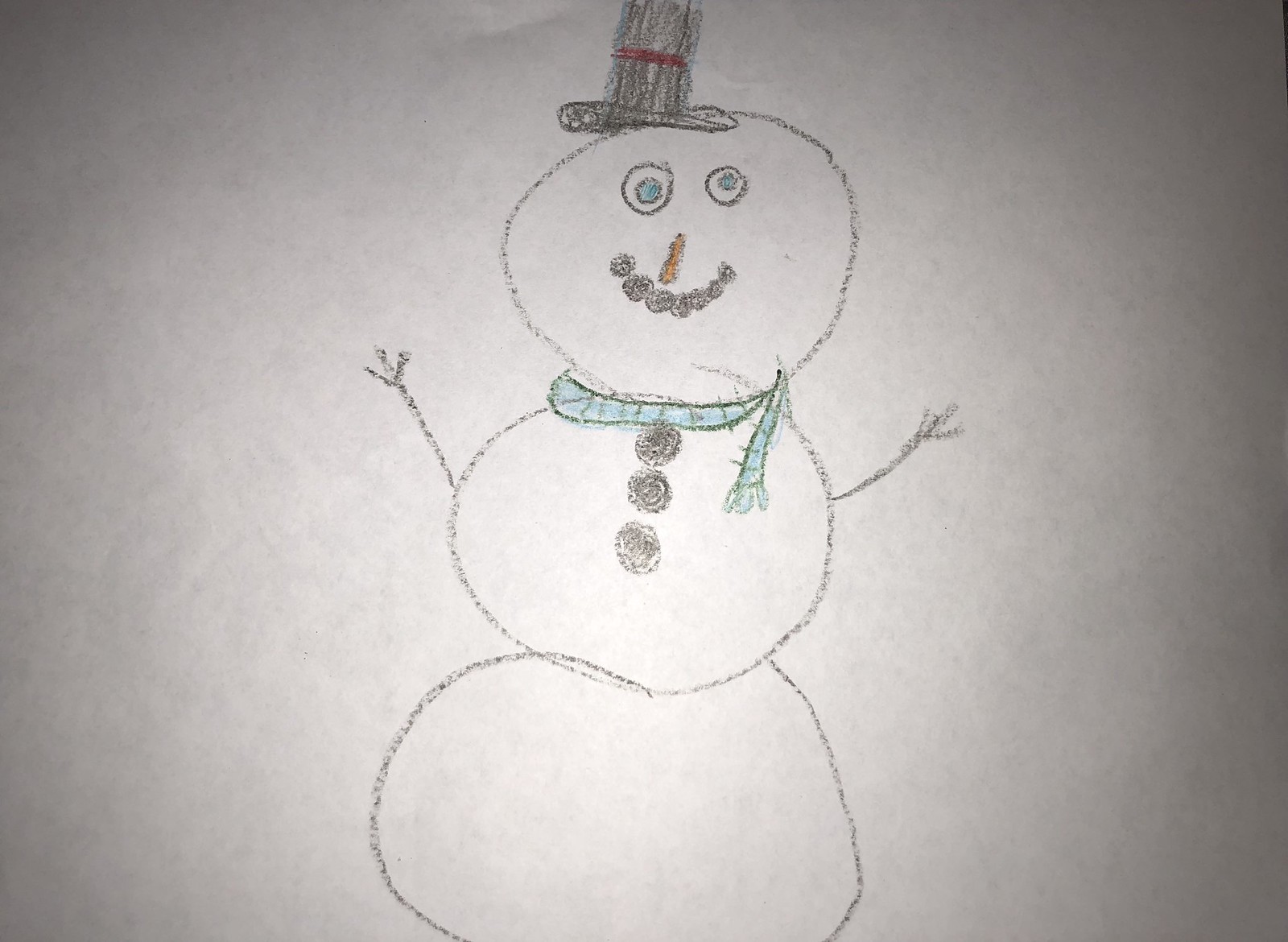This image showcases a charming, childlike drawing of a snowman set against a gray background, meticulously rendered using colored pencils. The snowman features a three-tiered body with imperfectly shaped ovals, suggesting the artistic hand of a young child. The middle section of the snowman is adorned with a line of three buttons running vertically down its front. A vibrant blue scarf with detailed lines denoting its fabric texture is draped around the snowman's neck, with one end stylishly flipped over the front of the second oval. 

The snowman's arms are depicted as stick branches, each extending from the middle section of the body and ending in three twig-like fingers. The head of the snowman bears six irregularly shaped dots forming a whimsical smile. A small, stick-like carrot signifies the nose, while the eyes are unique in their design—crafted as black circles filled with blue centers, with the right eye noticeably smaller than the left. Atop the snowman's head rests a classic black top hat, completing its endearing wintery appearance.